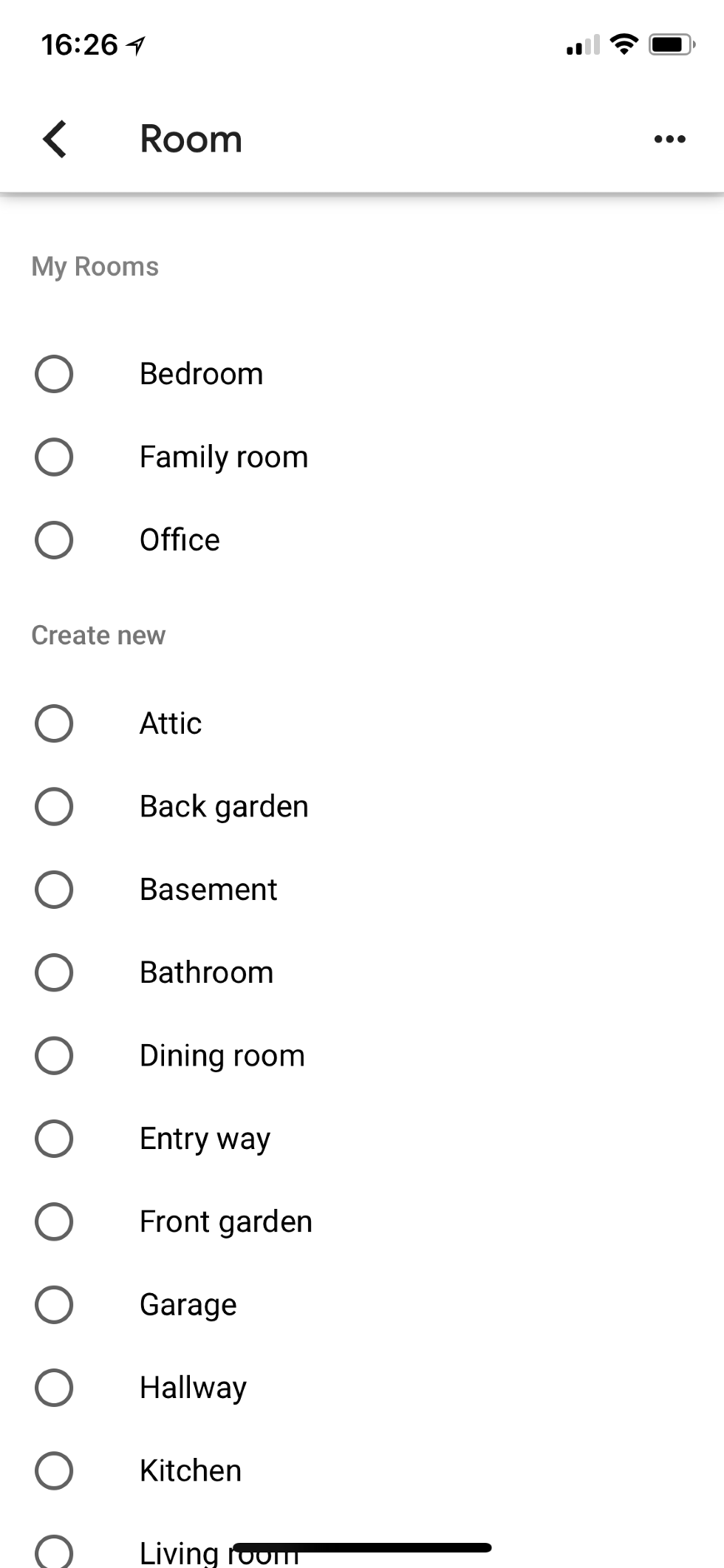A screenshot displayed on an iPhone presents a detailed interface related to room management or customization. The status indicators at the top of the screen show an iPhone with a nearly full battery and a strong internet connection, marked by two out of four signal bars. The current time reads 16:26.

At the top of the screen, a header reads "Room," accompanied by a left-facing arrow and three dots positioned on the right side of the header bar. The main section of the interface lists various rooms, divided into two sections titled "My Rooms" and another unnamed category, each room beside a hollow circle indicating a selectable or actionable item. The "My Rooms" section includes entries for "Bedroom," "Family Room," and "Office." Below this, a smaller font option reads "Create Room."

The unnamed category under "Create Room" lists additional locations such as "Attic," "Back Garden," "Basement," "Bathroom," "Dining Room," "Entryway," "Front Garden," "Garage," "Hallway," "Kitchen," and "Living Room," each with a corresponding hollow circle, suggesting interactive checklist options.

The purpose of the interface remains unspecified within the image, leaving it unclear whether it’s intended for constructing, painting, organizing, or another function related to room management.